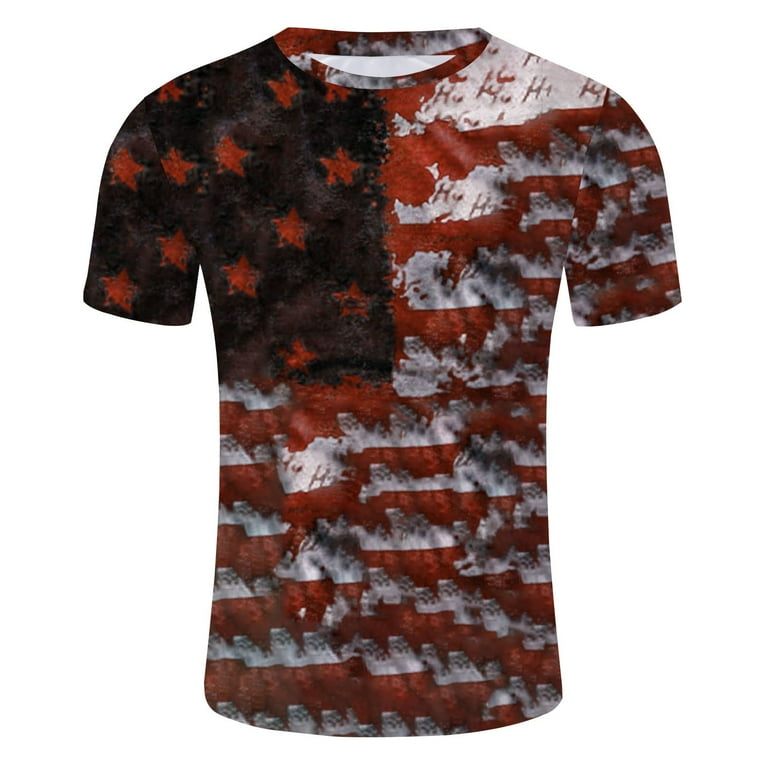The image features a distinctive short-sleeved, crew neck t-shirt inspired by the American flag. The design presents a rugged, abstract interpretation of the flag’s elements. The main body of the shirt, along with the left sleeve, is adorned with uneven and mottled red and white stripes that resemble sponge painting or stamp printing. These stripes are not straight but appear rugged and cloud-like, with red splatters subtly integrated into the white areas.

On the upper right side of the shirt, encompassing the right shoulder and sleeve, there's a dark background, possibly black or a dark blue-gray, covered with red stars. This section is set in a square pattern, providing a stark contrast to the rest of the design. Despite the abstract, uneven paint strokes and subdued tones, the shirt unmistakably echoes the American flag's patriotic vibe. The t-shirt is displayed against a white background, giving it a rounded appearance as if it’s being worn, although no mannequin is visible in the photo.